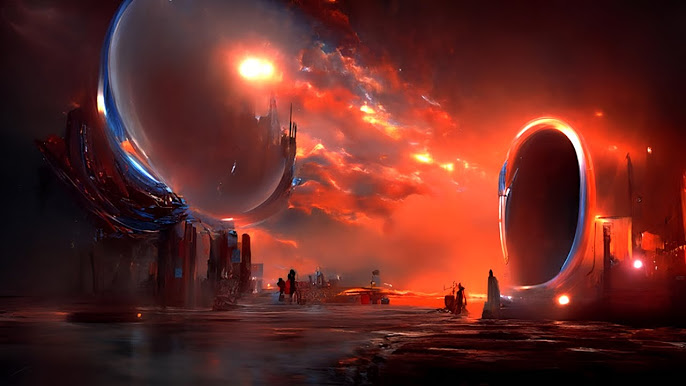The image is a digitally created futuristic illustration, marked by a strikingly red and smoky atmosphere that gives a sense of a surreal, otherworldly landscape. Dominating the right side is a large, vertical structure with a huge, wide-open mouth-like opening that reaches upwards, resembling a building or a tunnel. The ground is predominantly red, blending from what appears to be wet, reflective surfaces to more solid ground, and scattered with glowing lights. 

In the upper left portion of the sky, maroon and red hues resemble a sky on fire, with a semi-transparent orb-like bubble containing the faint outline of a castle. Behind this orb is a bright light source, akin to the sun, which casts a glowing orange haze throughout the central portion of the sky, dense with red, blue, and pink clouds. A distinct blue, glowing line borders the left side of this orb. Another similar yet vertical orb with a neon border sits on the right, contrasting against the darker landscape.

Amongst this fantastical scene, a few human figures can be seen walking around in silhouette, their attire indistinguishable, adding a sense of scale and mystery to the complex, undefined setting. The entirety of the scene captures the essence of digital fantasy space art, combining elements of science fiction with a vivid and arresting color palette.